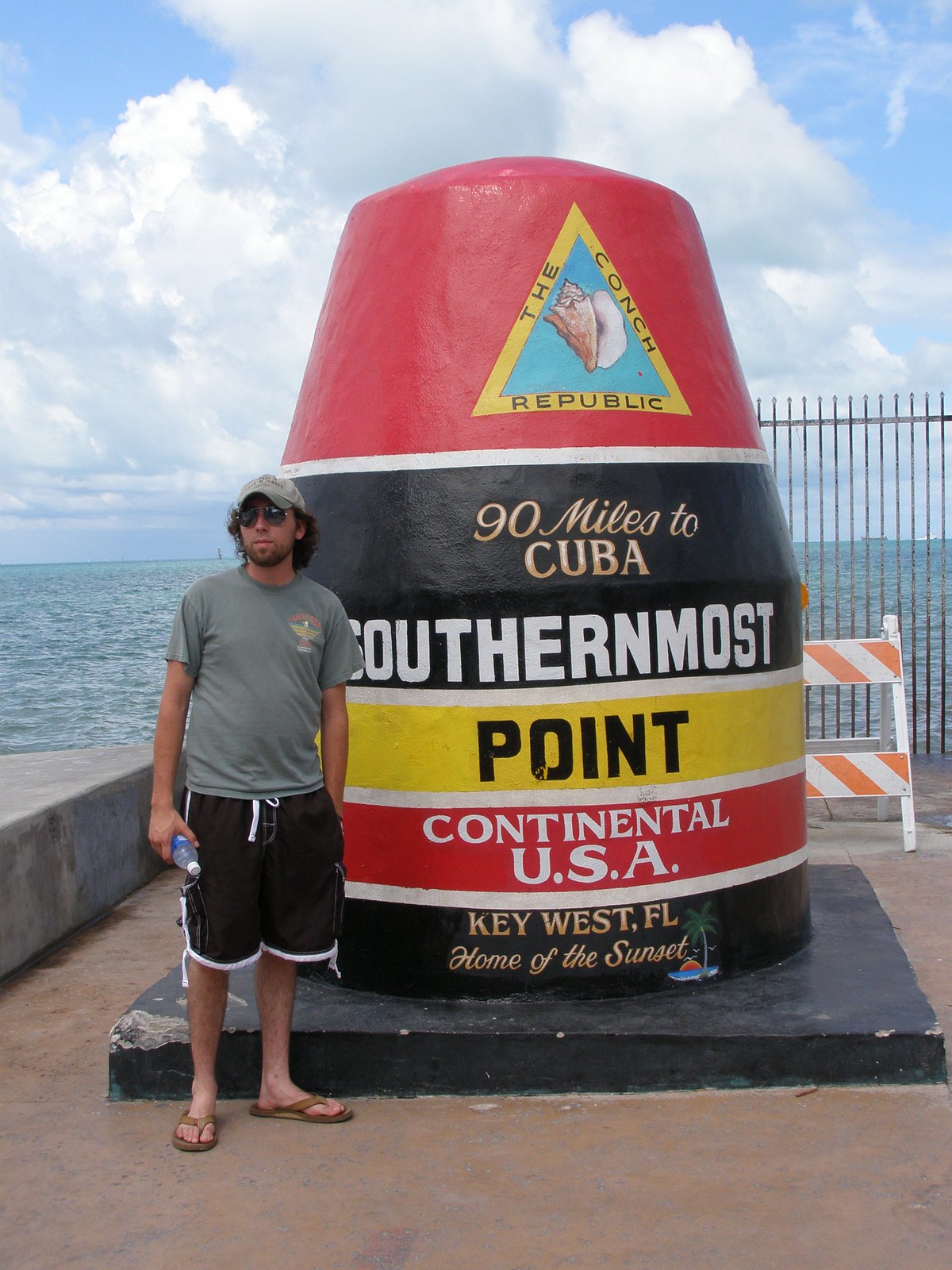In the photograph taken outdoors, a man stands in front of a prominent monument. The monument resembles a buoy, roughly 10 feet high, with alternating stripes of red, black, and yellow. At the top, there's a conch shell design and the words "The Conch Republic" above a yellow triangle. Prominently displayed text reads, "90 miles to Cuba, Southernmost Point, Continental USA, Key West, Florida, Home of the Sunset."

The man, who likely has brown hair and a beard, wears a tan baseball cap, dark sunglasses, a gray t-shirt, and black shorts with white trims, accompanied by tan sandals. He holds a water bottle in his left hand. Behind him, a high black metal fence borders the area, beyond which the open ocean stretches outward with islands faintly visible on the horizon. The sky above is partly cloudy, featuring big, puffy white clouds with patches of blue peeking through. The scene is serene but slightly dreary, capturing the essence of a cloudy day by the water.